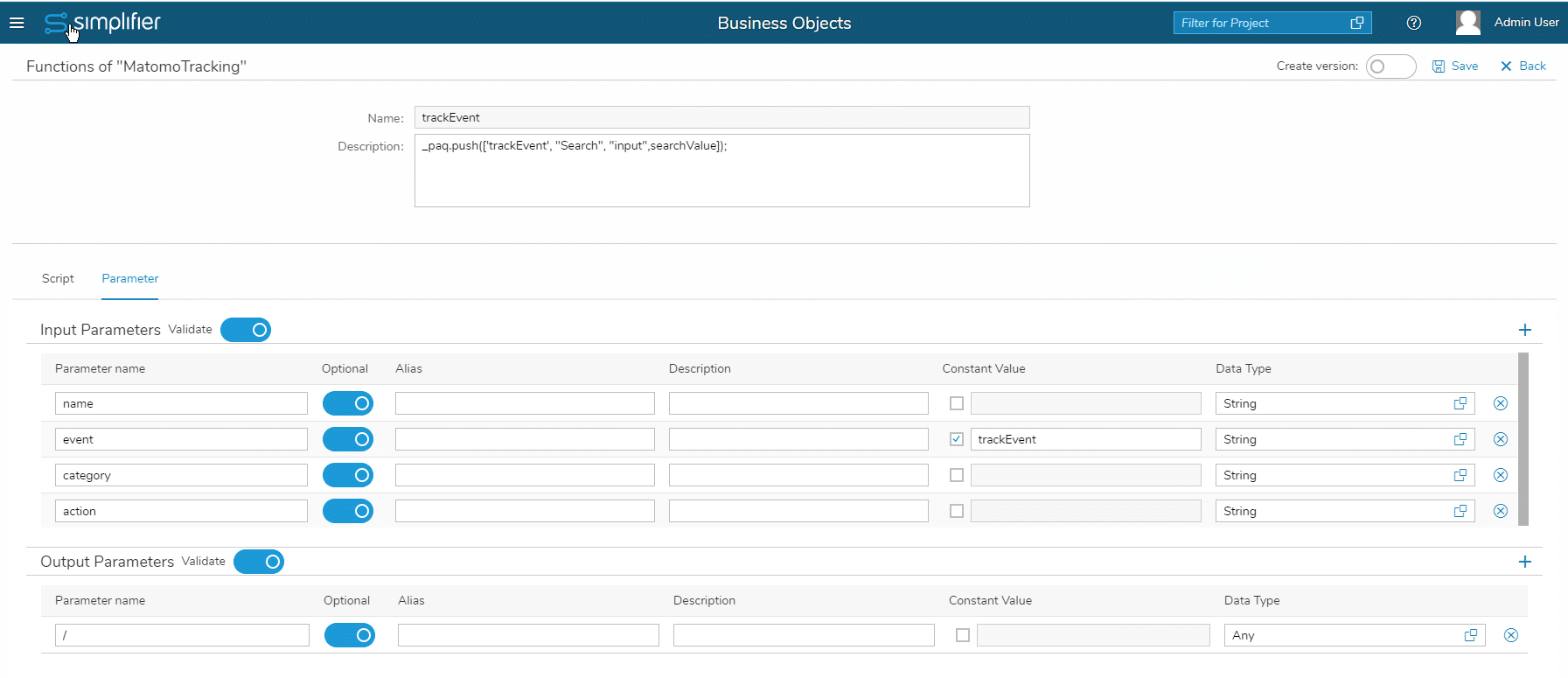In the screenshot, a prominent bluish-gray bar spans the top from left to right. On the left, there are three horizontal white lines indicating a menu, followed by a logo resembling an 'S' with a dot at each end. To the right of this logo, the text "Simplifier" is displayed, with the 'S' in blue and the remainder in white. Centrally positioned in white text, it says "Business Objects." Further to the right, a white text box labeled "Filter for Project" is visible, accompanied by two white rectangles, a question mark icon, a blank picture icon, and the text "Admin User."

Beneath the blue bar, against a white background, there are gray text headers and fields. The title "Functions of Maximal Training" is displayed in gray. In the central section, there are two prominent text boxes: the first labeled "Name" with "Track Event is written," and the second labeled "Description" with the content "_PAQ.push("Track Event", "Search", "Input", "SearchValue")."

To the right, an unfilled toggle for "Create Version" is visible, alongside a disk icon labeled "Save" and an 'X' icon labeled "Back."

Under these elements is a separator line followed by two sections labeled "Script" and "Parameter" in black. The "Script" section includes an input field and a blue-selected "Validate" toggle. The "Parameter" section features headings like "Parameter Name," "Optional," "Alias," "Description," "Concept Value," and "Data Type." Several lines have text entries, toggles, checkboxes, and copy icons. Specifically:

- Parameter rows: 
  1. Name: "Name" with a blue toggle.
  2. Event: "Event" with a blue toggle.
  3. Category: "Category" with a blue toggle.
  4. Action: "Action" with a blue toggle.

Only the "Track Event" checkbox is marked under "Concept Value," written in camel case (TrackEvent). Data Type for all parameters is "string," each followed by a copy icon and a blue circle with an 'X.'

At the bottom, the "Output Parameters" section mirrors the input parameters layout: "Parameter Name," "Optional," "Alias," "Description," "Concept Value," "Data Type," with an initial entry having a slash ('/') and a toggled-on switch labeled "Validate." All subsequent fields are largely blank, once more with copy icons and 'X' symbols, finishing with Data Type marked as "Any."